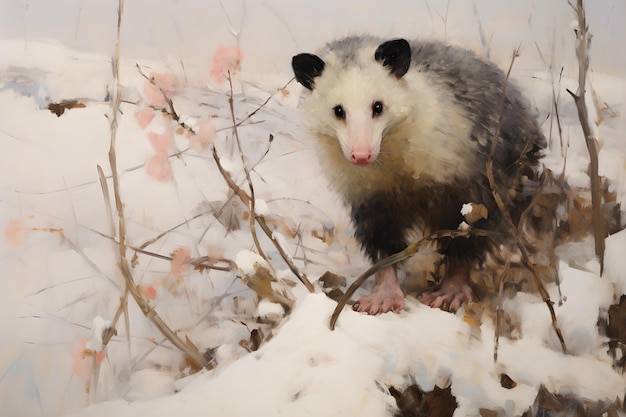This detailed hand-painted image on canvas beautifully captures a lone opossum in a snowy, arctic tundra scene. The opossum, with its distinctive pink nose and black ears, has intricately rendered fur showcasing subtle shades of brown and hints of golden highlights beneath its neck. Its beady black eyes sparkle slightly, adding an expression of curiosity as it faces forward. The creature stands amidst a picturesque winter landscape of snow-dusted twigs, branches, and bushes adorned with delicate pastel blossoms. The background is a stark, nearly white skyline, enhancing the cold, serene ambiance of the scene. Each brush stroke meticulously portrays the texture of the opossum’s fur and the surrounding natural elements, reflecting the artist’s attention to detail and skill.